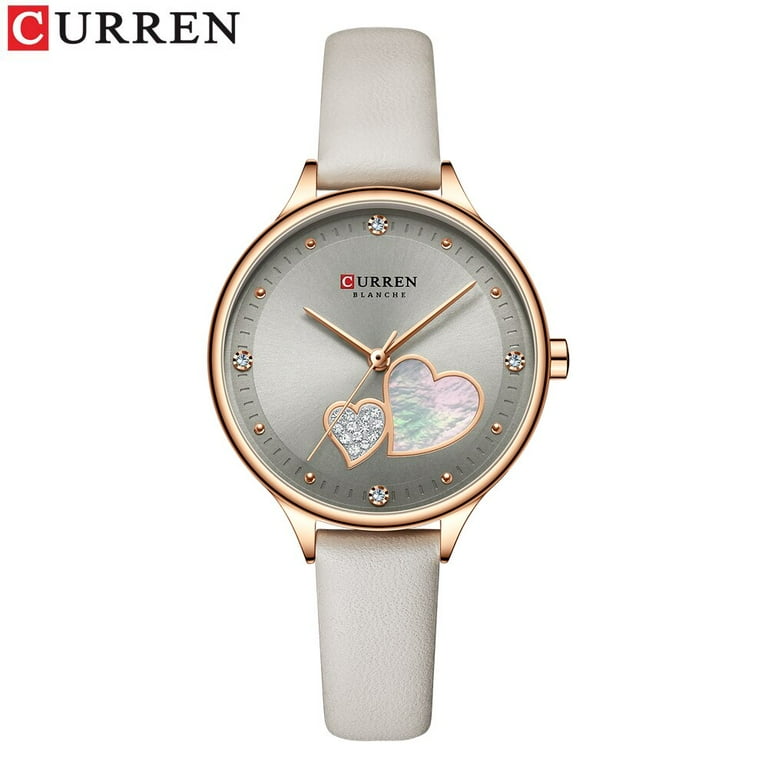This advertisement is presented in a rectangular, portrait-oriented format. Positioned in the upper left-hand corner is the brand name "Curran." The design of the lettering features a white 'C' against a bold red background, while the remaining letters "urran" are displayed in a sleek black font. Central to the advertisement is a striking photograph of a wristwatch. 

The watch boasts a light gray band, exuding a modern yet classic elegance. Encircling the face of the watch is a sophisticated rose gold border that enhances its luxurious appeal. The watch face is marked with the branding "Curran Blanche," offering a sense of exclusivity and style.

Adding a touch of charm, two delicate heart symbols adorn the lower portion of the watch face, symbolizing love and attention to detail. The current time displayed on the watch reads 10:08, captured in a clear and precise fashion. This polished presentation effectively showcases the elegance and sophistication of the Curran Blanche timepiece.